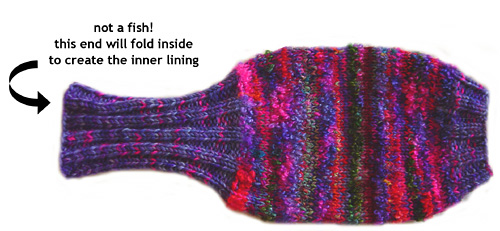The image features a uniquely knitted textile piece that resembles a sock but is not. Multicolored with hues of blue, pink, green, purple, red, and a hint of orange, the item is vibrantly crafted with an abstract design. The textile is shaped somewhat like a fish or a vase, with narrower ends and a wider middle section, illustrating an intricate design. An arrow pointing to the smaller end of the item highlights a caption in small black letters stating, "Not a fish. This end will fold inside to create the inner lining." The piece appears soft and elastic, with possible uses inferred but not definitively identified—potentially suggested as part of a sweater or even a boot lining. The background of the photo is a plain, clean white, providing stark contrast to the colorful textile.